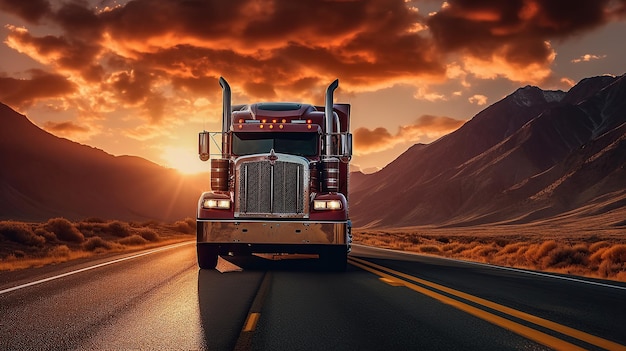The image depicts a dynamic, vividly colored painted or drawn scene of a large maroon 18-wheeler truck, or big rig, driving directly towards the viewer. The truck is centered on the road, straddling a single dashed yellow line, with a solid double orange line visible to the viewer's right. The truck features distinctive dark-tinted windows, making it impossible to see the driver, and is outfitted with two prominent smokestacks on either side of the windows. Its headlights are on, illuminating the road ahead.

The surrounding environment is quite dramatic, with the scene set during either sunrise or sunset. The sky is filled with a striking blend of colors – heavy clouds at the top that fade into a vibrant orange at the bottom, and the sun itself, a bright yellow orb, peeks through, casting an orange glow across the landscape. The asphalt road is flanked by grass similarly bathed in the orange light, and mountains frame both sides of the scene, suggesting the truck is navigating through a valley. The attention to detail in the painting highlights the silver bumper, black tires, and the overall imposing presence of the big rig as it progresses down the highway.